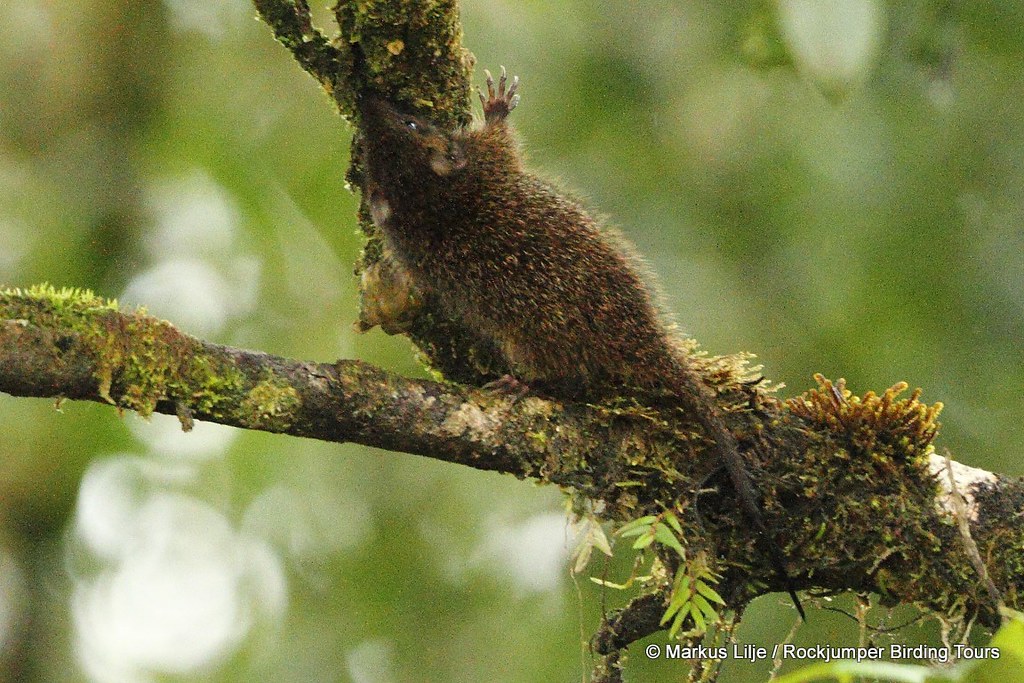In this image captures an intricately detailed scene of wildlife, focusing on a small baby squirrel, which exhibits some unique rodent-like characteristics. The squirrel, with its dark brown head and a brown body interspersed with golden, black, and yellow hairs, is in the process of crawling up a vertical branch, reaching towards a higher point with its hand-like claws that have five white-tipped fingers. The squirrel's tail is thin and extends into a sharp point. 

The branch, adorned with moss-like grass ranging from green to gold colors, extends from the bottom left-hand corner of the frame diagonally towards the center. The background, a blur of varying shades of green and white, suggests a forest setting, although it remains unfocused to emphasize the main subject. The squirrel's back is turned to the camera, giving a sense of movement and determination as it navigates its arboreal environment. At the bottom of the image, there is a line of text that reads "Marcus Rockjumper Birding Tours," adding a subtle context to the serene yet dynamic wildlife scene.